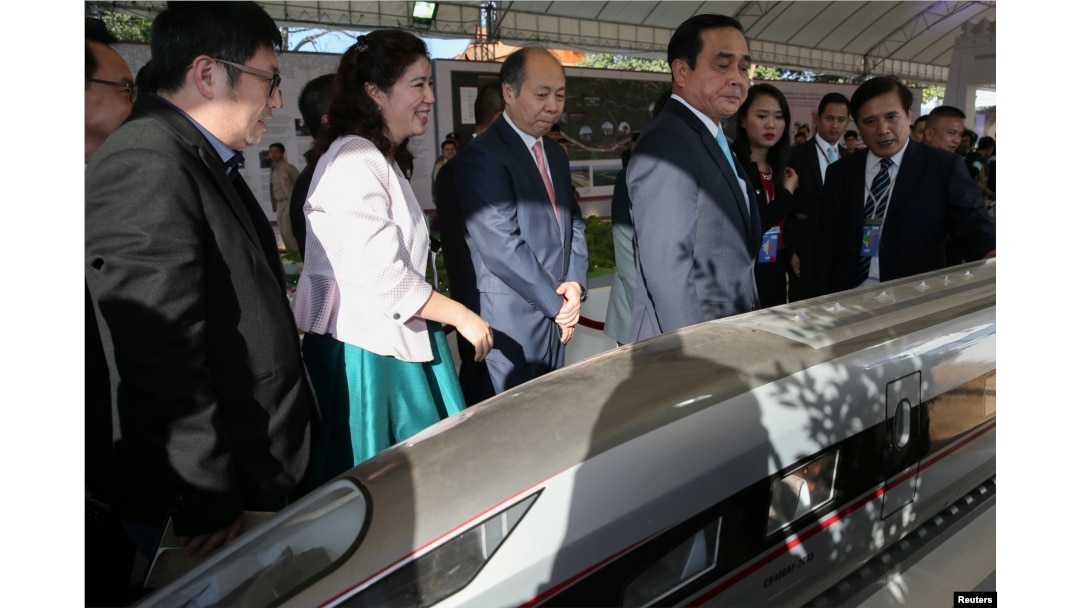In this image, a group of people of Asian descent are gathered in an open sheltered area, likely a pavilion or exhibit space. They are standing at a railing, appearing to be closely examining a detailed model of a modern bullet train. The train has a dark gray top, lighter gray sides, and features a distinctive black and blue stripe along its bottom edge, with shadows that cast interesting patterns around it. 

Starting from the left, there is a man in a black coat with black hair and glasses. Next to him is a smiling woman with black hair, wearing a pink suit paired with a teal dress and holding one hand forward. Beside her stands a balding man in a dark blue suit with a red tie. To his right, a man in a black suit with neatly styled black hair is looking intently at the train. At the end of the row is another man in a dark suit and tie, with a white lanyard and blue tag around his neck, also focused on the model. The display area appears to have framed posters or panels behind the group, adding context to the exhibit they are reviewing.